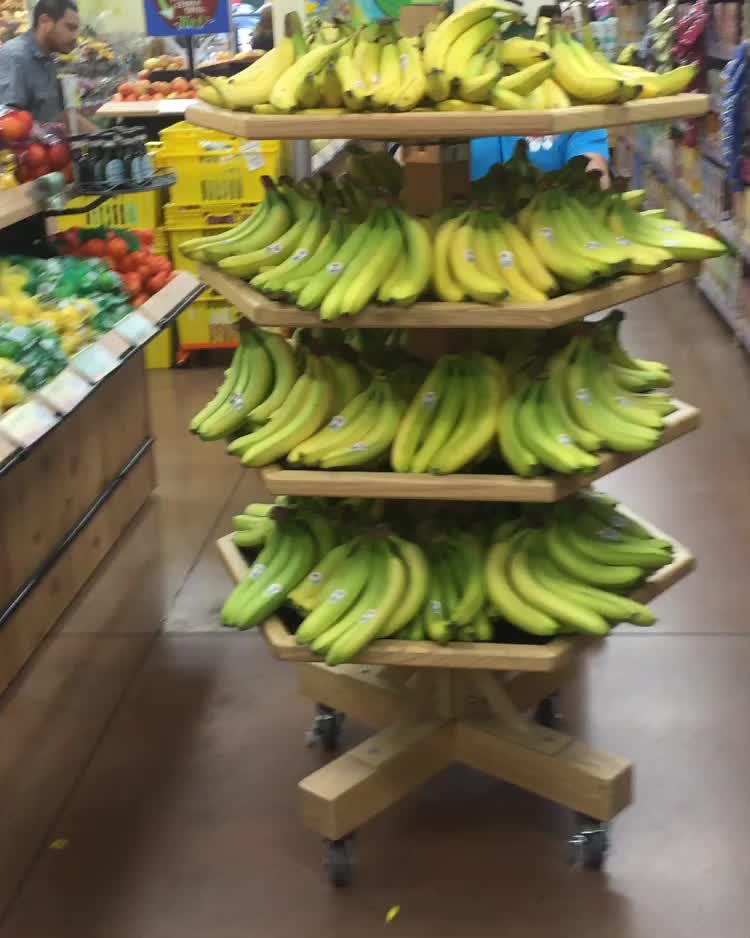This photograph captures a bustling scene in a grocery store's produce section. In the center of the image, there is a distinctive wooden display stand with wheels, designed with hexagonal layers stacked vertically. Each of the four hexagonal shelves is laden with bunches of bananas, creating a tiered arrangement. The bananas on the lower shelves are predominantly green, while those on the top shelf are the most yellow, indicating different stages of ripeness. To the left of this central banana display is another produce shelf featuring a mix of fruits including oranges, tomatoes, lemons, and limes, with the upper part of the shelf only partially visible. Further to the left, near some yellow crates, a person is seen from the chest up, seemingly inspecting the produce. To the right, a wall is lined with various products in colorful blue and red packaging, although the exact details are obscured by the photo's low quality. Another person in a blue shirt can be seen behind the banana stand, their arm outstretched, possibly reaching for a bunch of bananas. The store floor is a brown color, grounding the scene in a warm, earthy tone. The overall image is slightly fuzzy but clearly shows the vibrant and busy environment typical of a grocery produce section.